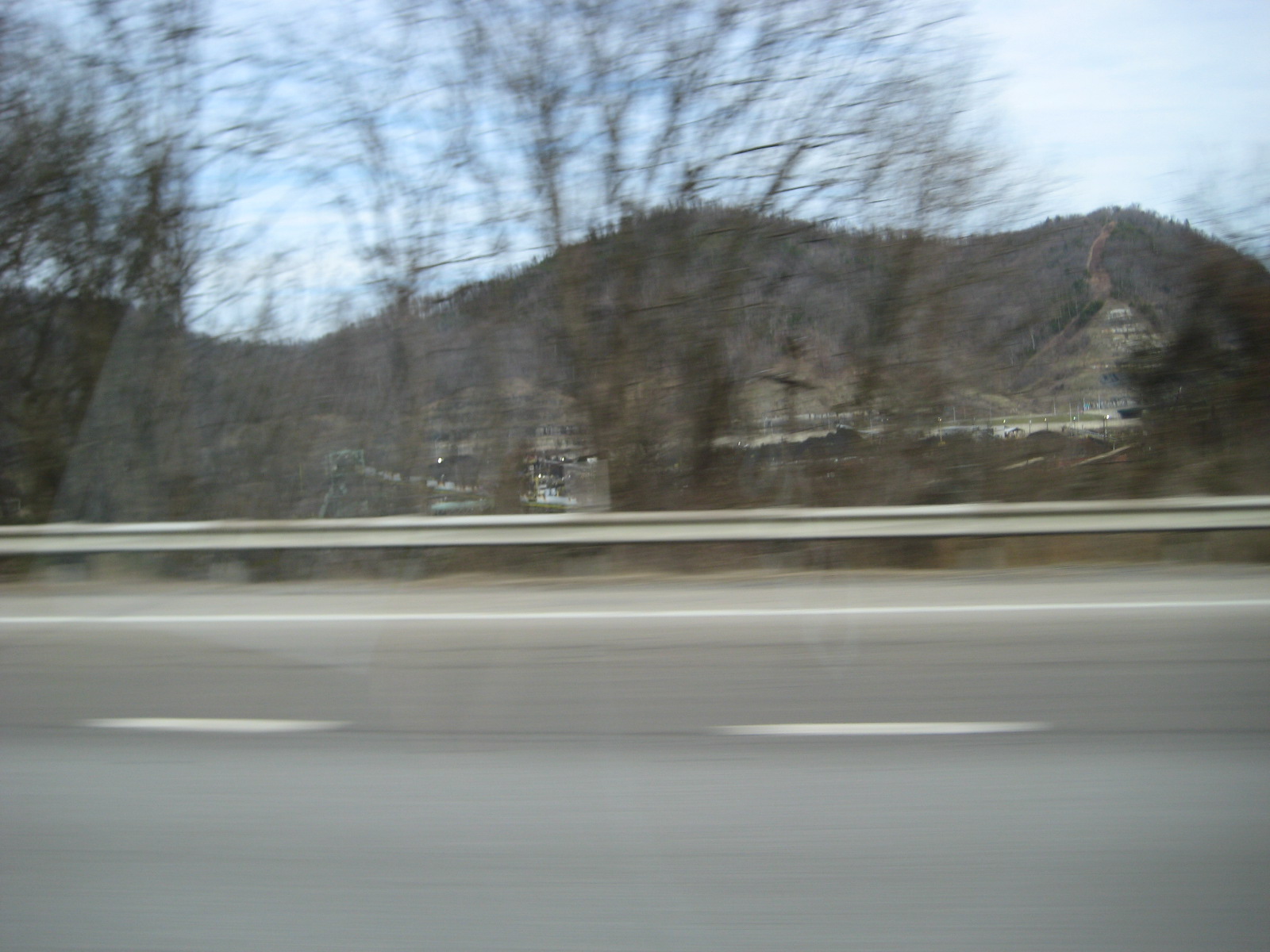The image appears to be a motion capture photograph taken from inside a moving car, possibly during winter. It showcases a stretch of empty paved highway marked with white lane separators. Running along the edge of the road is a steel guardrail. Beyond the guardrail, barren and leafless trees suggest a cold season. In the background, an expansive valley can be seen, with a silhouette of hilly terrain covered in sparse vegetation outlined against the pale blue sky. The landscape includes a town with numerous buildings nestled at the base of the hills, with more structures visible on the slopes. A visible pathway snakes up the right side of the tallest hill, leading to additional buildings at higher elevations. The reflection in the car's window hints that the photo was taken by a passenger.